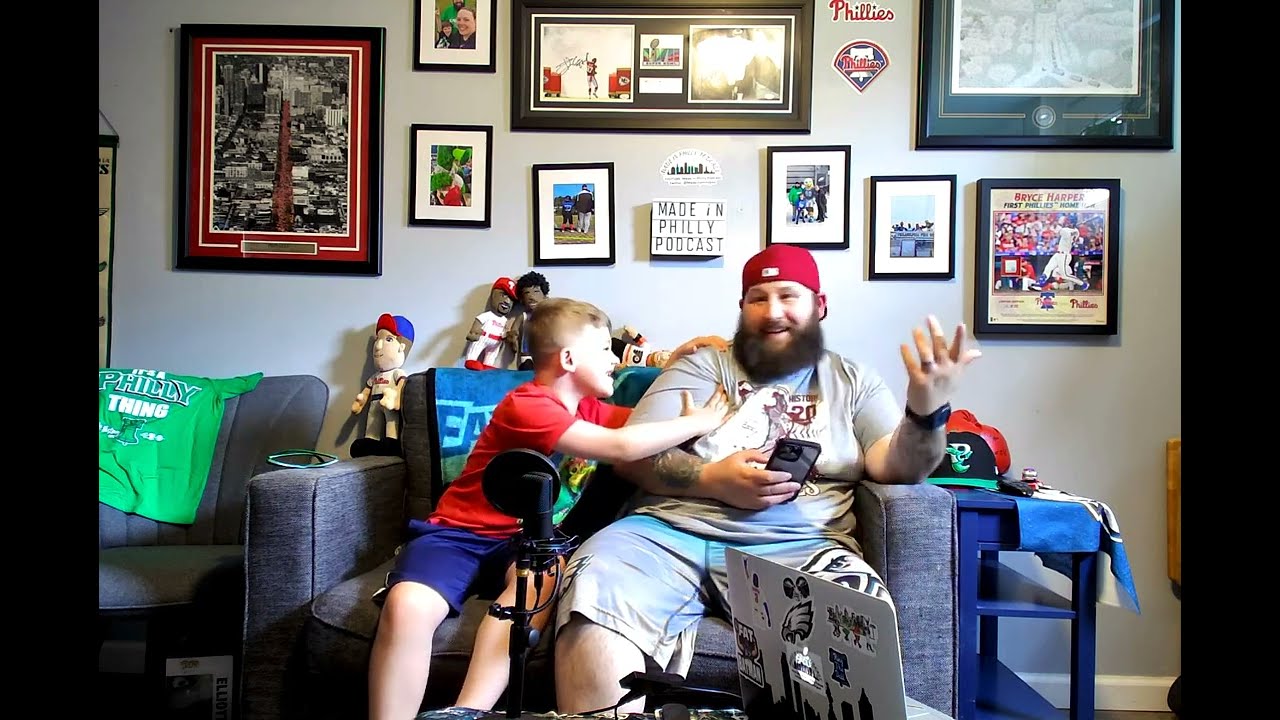A picture captures a moment between a bearded man and a young boy, who appear to be father and son, sitting on a gray two-person couch in a room adorned with Philadelphia sports memorabilia. The man, sporting a white t-shirt with a possible baseball logo, jean shorts that extend over his knees, and a backward red baseball cap, is engrossed in his cell phone. The boy, dressed in a red t-shirt and blue shorts, is affectionately leaning on or playfully pushing his dad. Surrounding them are various baseball bobbleheads and sports memorabilia, including posters of Bryce Harper and signs that say 'Made in Philly Podcast,' suggesting the man may be a podcaster focused on Philadelphia sports. A green shirt draped over a gray chair reads 'Philly Thing,' further emphasizing their Philly pride. In the foreground sits an open laptop, adorned with Philadelphia-related stickers, along with a microphone, hinting that they might be recording a podcast together. The wall behind them is filled with photos, frames, and posters, creating a vibrant backdrop that underscores their shared love for Philadelphia sports.